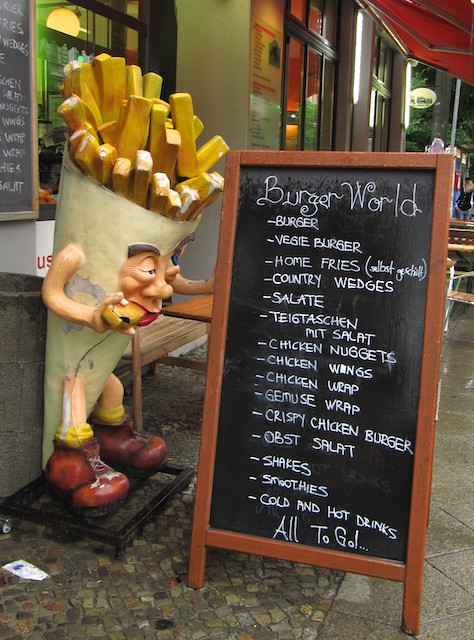Outside of a restaurant, there's an eye-catching display that features a large, charmingly eccentric statue and a detailed chalkboard menu. The statue, perched on the left, is a quirky anthropomorphic cone of French fries. It depicts a small, leprechaun-sized figure with a jovial face, complete with one squinted eye and one open eye, a prominent nose, and lips emerging from the cone. The fries at the top mimic the character's hair, while its yellow socks and brown (or dark red) shoes add to its whimsical appearance. The statue appears to be munching on a fry taken from its own head, adding a playful touch to the scene.

Next to the statue is a chalkboard sign with a standard wooden border, displaying the restaurant's offerings in white chalk against a black background. The top of the board features the restaurant name "Burger World" in large, squiggly font. Beneath it, a variety of menu items are listed, including:
- Burger 
- Veggie Burger 
- Home Fries 
- Country Wedges 
- Salad 
- Chicken Nuggets 
- Chicken Wings 
- Chicken Wrap 
- Crispy Chicken Burger 
- Wrap options: Gamuse Wrap, T-gueskin, and Mitzpat
- OBS Tea 
- Shakes 
- Smoothies 
- Cold and hot drinks

At the bottom of the chalkboard, it emphasizes that all items are available "to go" with a playful exclamation point and ellipsis.

Both the statue and the sign rest on a cobblestone surface featuring a mix of grayish-brown stones of various colors. The setting, with its multiple windows, doors, and a red awning that stretches over the front entrance, suggests a welcoming and casual atmosphere for diners.